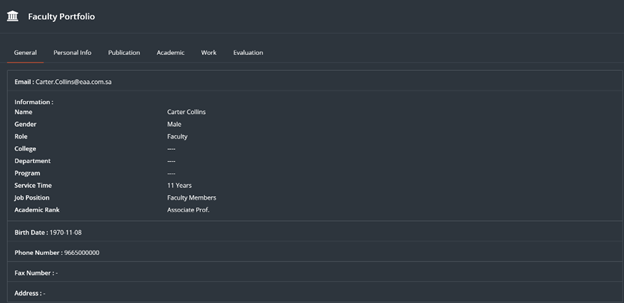Screenshot of a Faculty Portfolio Website

This image showcases a screenshot from a faculty portfolio website, specifically highlighting the general settings section. At the top, the primary contact email is listed, addressed to Carter Collins. Following the email, detailed personal information about Carter Collins is presented. He is identified as a male faculty member with a role in academia. Collins has accrued 11 years of service, holding the position of an associate professor. Additional details include his full name, birth date, and phone number. Notably absent from the screenshot are his fax number and physical address.

Adjacent to the "General" settings subtitle, there are several other tabs labeled "Personal Info," "Publication," "Academic," "Work," and "Evaluation." These tabs suggest that the website provides comprehensive information regarding Carter Collins' professional and academic contributions, as well as personal details relevant to his faculty role.